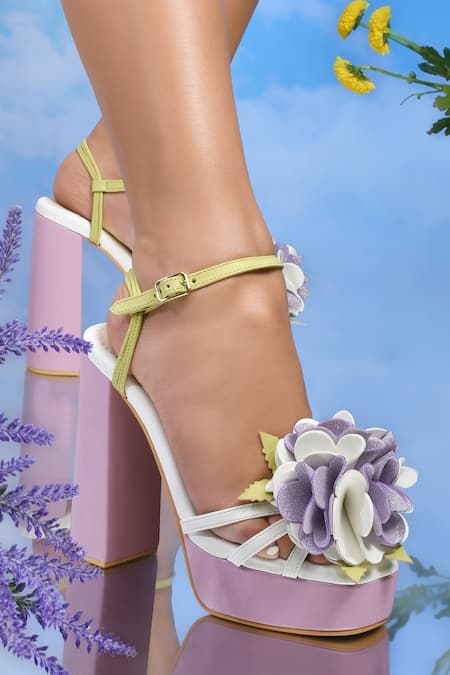This close-up, angled photo captures a woman with bronze skin and white manicured nails, showcasing a stylish high-heeled platform shoe. The shoe features a thick heel and a vibrant combination of colors. The bottom of the high heel is purple with a golden sole, and it is adorned with a white strappy front. An ankle strap, colored in gold, secures the shoe, which also sports a purple and white flower with green leaves and a small gold buckle on the side of the strap.

The woman stands on a shiny, reflective blue surface, which mirrors the image of the shoe, adding depth to the scene. To the left of the image, lavender flowers encroach into the frame, and in the top right corner, three yellow flowers, resembling sunflowers or daffodils, add a touch of brightness against a backdrop that suggests a blue sky.